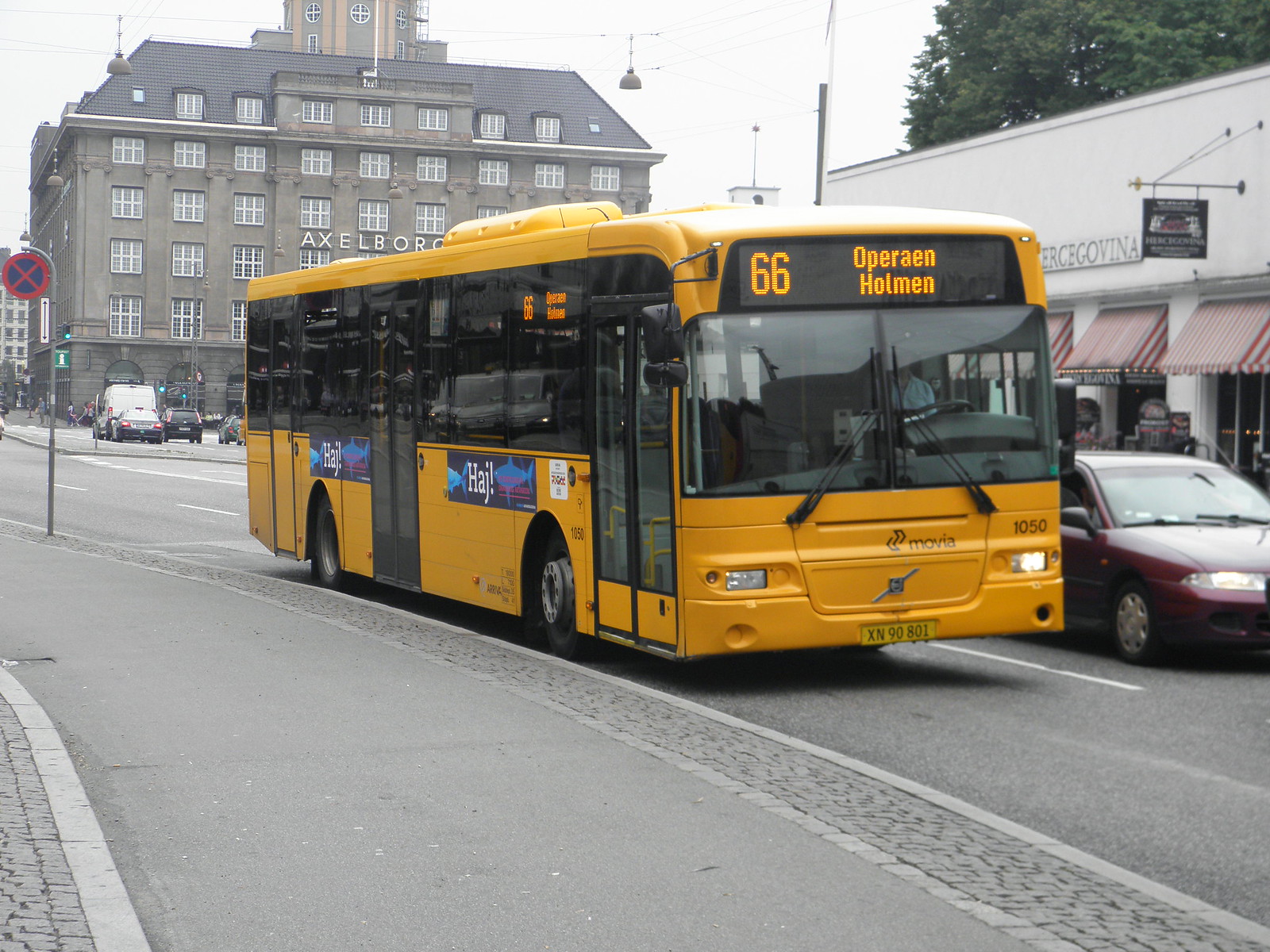In this detailed and colorful cityscape, the focal point is a bright yellow and black European street bus numbered 66, with a digital display reading "66 Operain Holmen." The bus is traveling towards the viewer along a gray cobblestone-lined road, with part of the road and sidewalk visible from the viewer's standpoint. To the right of the bus, a maroon sedan drives near a white building adorned with red and white striped awnings, hinting at a possible cafe or storefront. Above its windshield, the bus has large black windows and doors, with smaller blue advertisements on its side featuring shark illustrations and the word "Haj" in white letters. The bus itself is also marked by the word "Movia" and the number "1050" near the bottom.

In the background stands a large, multi-storied gray building with the letters "AXELBOR" prominently displayed, indicative of an old-style architectural structure, likely named Axelborg, situated in Copenhagen, Denmark. A tree canopy peeks through in the upper right, adding greenery to the urban scene. A circular traffic sign with a red X on a blue background mounted on a silver pole draws attention on the left side of the frame. The weather appears overcast, casting a soft light over the scene, enhancing the visibility of various elements such as the cobblestone street, vehicles, and architectural details.